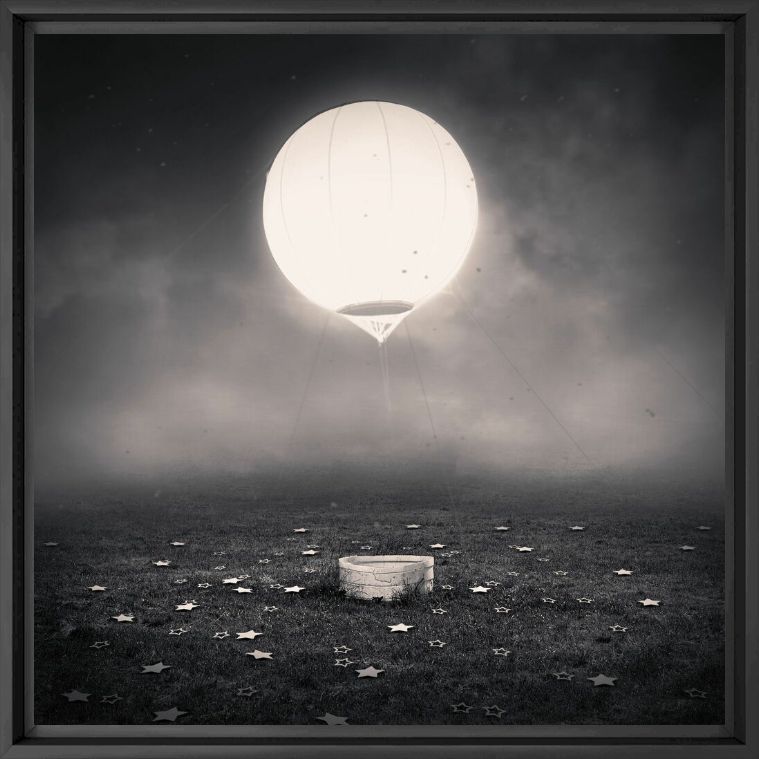In this black and white artwork, enclosed in a dark gray-colored frame with a subtler gray inner border, we observe a serene, surreal nighttime scene. At the center, there's a simple stone well surrounded by sparse gray grass. Sprinkled on the ground are small, hollow stars and larger, solid ones. Anchored above the well by guide wires, a hot air balloon glows with an intense white light, seemingly serving as the scene's solitary light source. The basket of the balloon rests gently on the ground, suggesting a mysterious, whimsical platform. The gray-hued sky is scattered with murky clouds, adding to the overall dreamlike, ethereal atmosphere of the artwork.